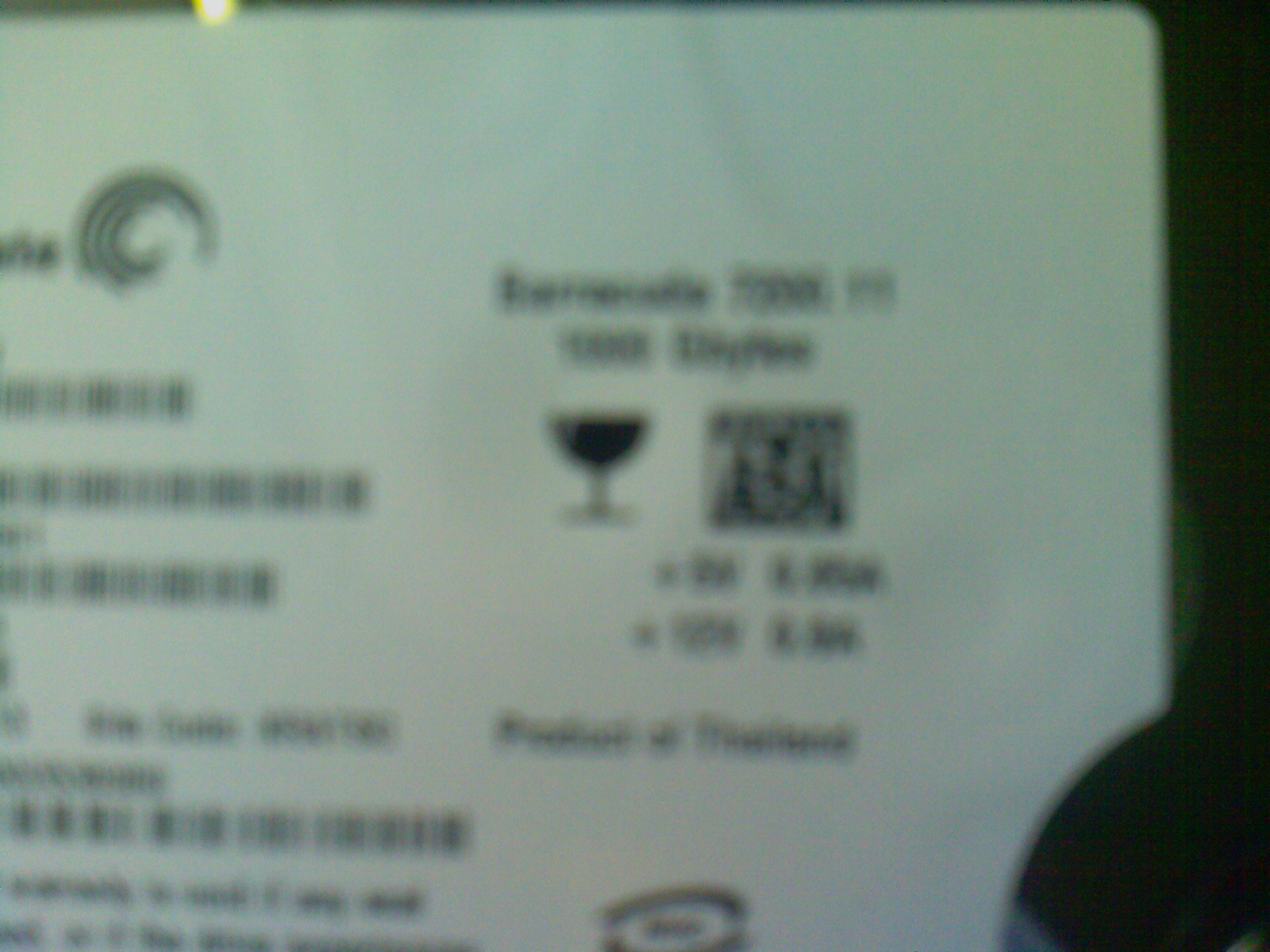This is a color photograph depicting what seems to be a section of a menu or poster, albeit out of focus, rendering the text illegible. The scene captures the top-right corner of the item, where two lines of type can be faintly seen. Adjacent to the text, there is a simplistic, black rendering of a wine goblet. To the right of the goblet, a blurry, unidentifiable logo appears, which consists of three lines at its center. The left side of the image features more blurred lines of text, topped with a swirl-like design element that adds a touch of decor to the otherwise indistinct visual.